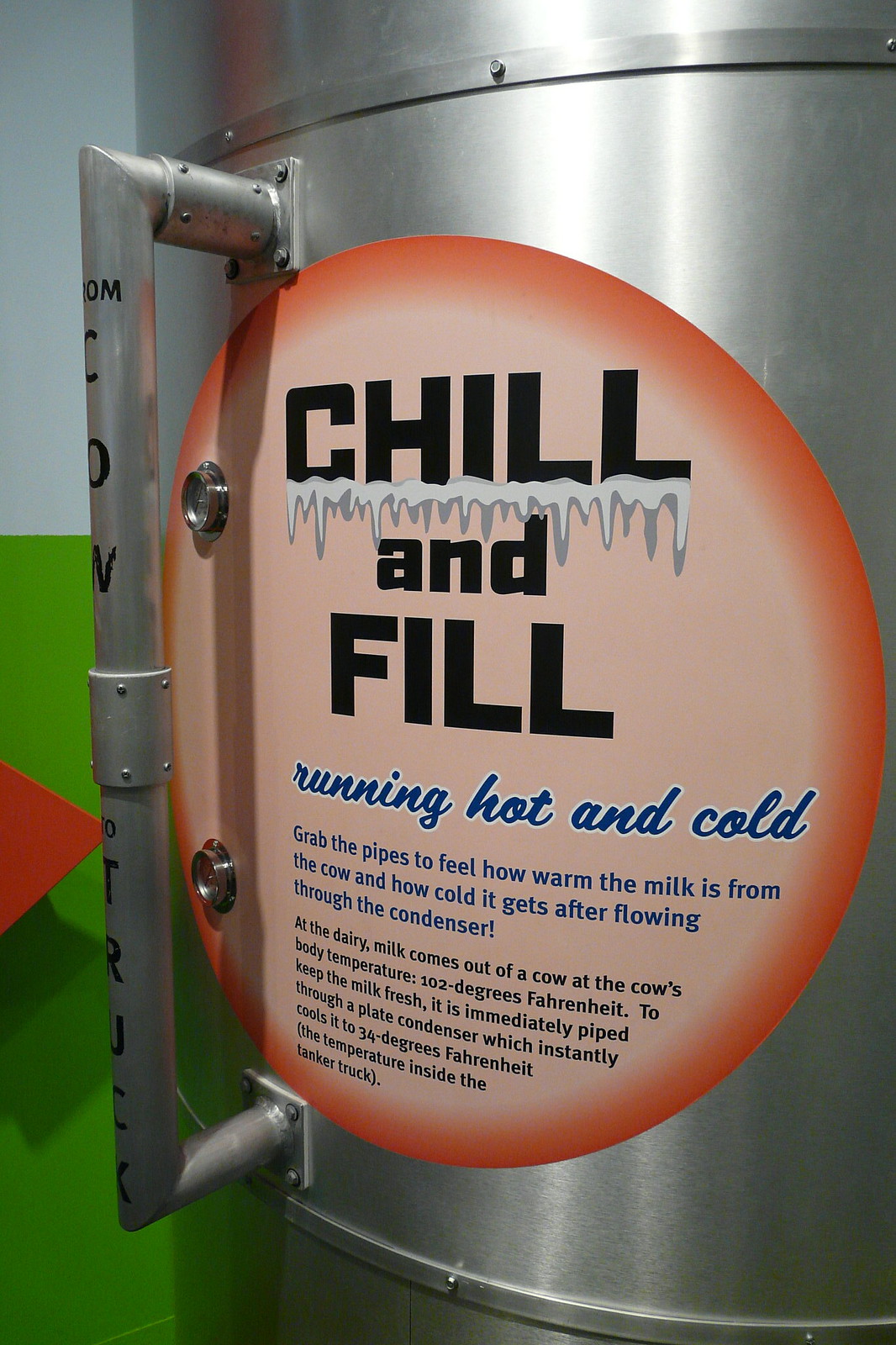The image in portrait view showcases a large silver vat, possibly part of a dairy or brewery's fermentation or cooling system. The vat's bottom, top, and right sides are cut off, but its reflective metallic surface catches the light predominantly on its top left. To the left of the vat, a handle-mounted bar, inscribed with black text, runs vertically and supports a prominent circular sticker. The sticker gradient transitions from a dark outer red to a lighter coral center, featuring the bold black uppercase text "CHILL AND FILL," with icicles hanging from the word "CHILL." Beneath this, in dark blue cursive, it states "Running hot and cold," followed by instructions in smaller black text: "Grab the pipes to feel how warm the milk is from the cow and how cold it gets after flowing through the condenser." Further details explain the milk's journey in the dairy process, indicating it is piped through a plate condenser instantly cooling it from the cow's body temperature of 102 degrees Fahrenheit to 34 degrees Fahrenheit, the temperature maintained inside the tanker truck. The background is divided into a top section of bluish gray and a bottom section of bright green, featuring a red triangle in the middle of the green expanse. This setting is illuminated, making the details and colors vivid and clear.